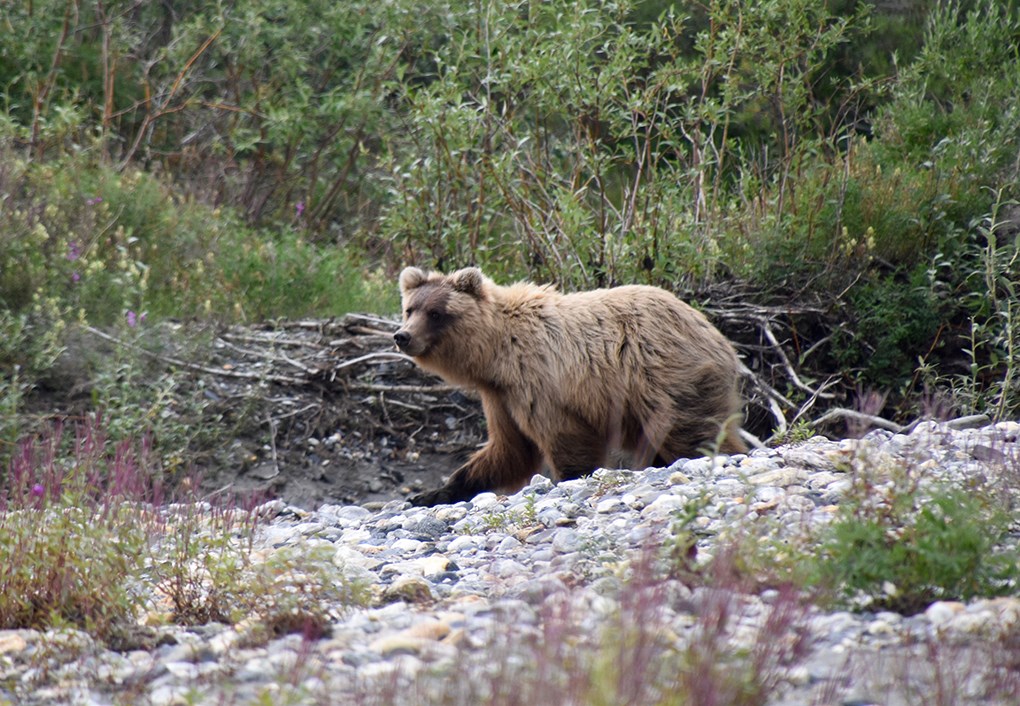This photograph captures a youthful, somewhat scruffy grizzly bear, most likely a yearling, perched on the edge of a creek. Although the creek itself isn't visible, the surrounding environment suggests its presence with round, river rocks spread across the foreground. The bear, with light brown and beige fur that darkens towards its legs and almost black paws, exhibits a noteworthy dark brown stripe along its face. It appears relaxed and seemingly unaware of the photographer, crouching slightly and staring intently, possibly towards the creek.

The background reveals a thick thicket of green bushes and timber, reminiscent of an Alaskan grizzly bear habitat ideal for salmon migration. Interspersed among the greenery are sporadic purple flowers, adding subtle hues to the predominantly green scenery. Stems and leaves dominate the backdrop, with branches and sticks forming a natural collage. The composition also includes a slight incline both in front and behind the bear, suggesting the variability of the terrain. This detailed scene captures the essence of untouched nature, with the bear as a focal point amidst a rich tapestry of bush and rock.